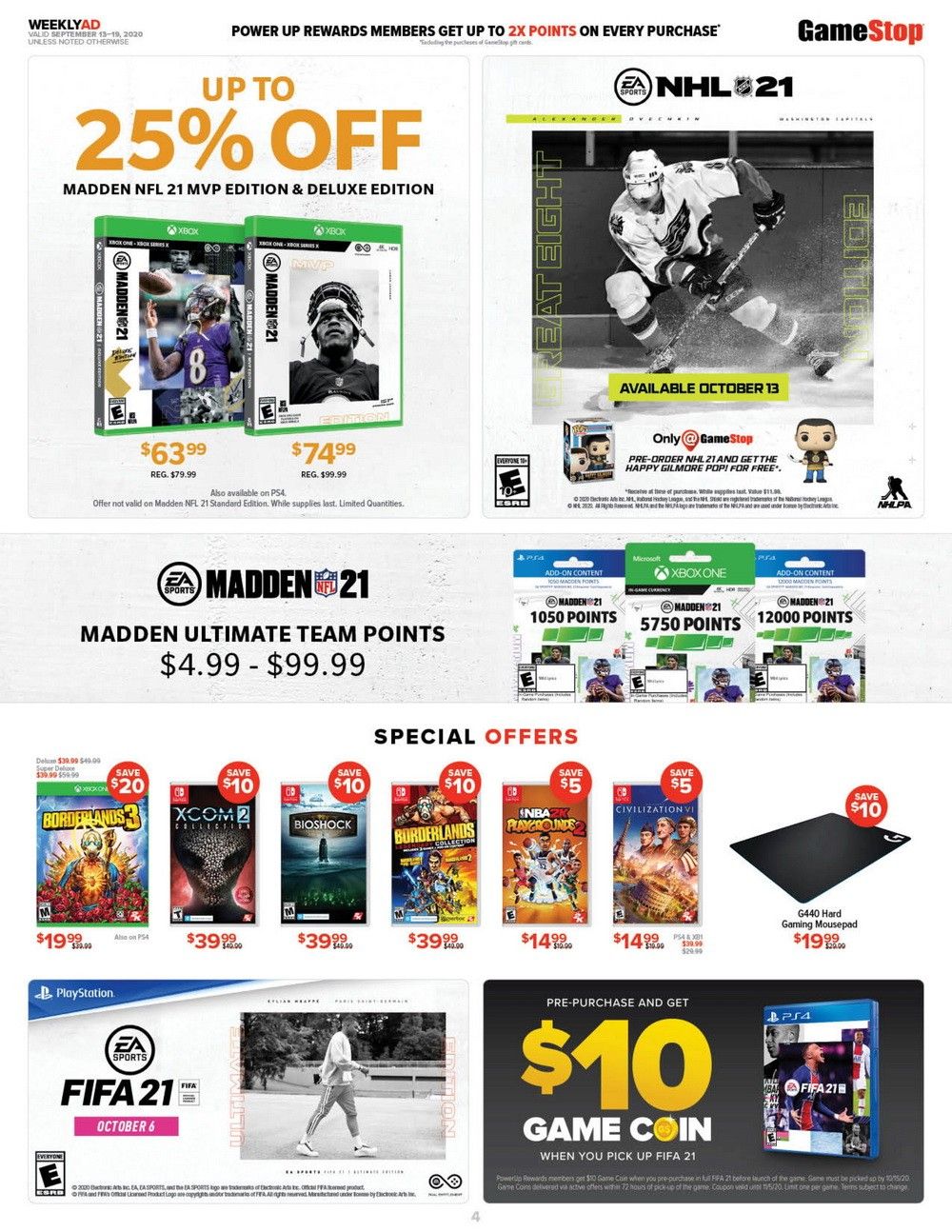This vertical, rectangular image is filled with sports-related promotional information. At the top left corner, it features the single word "weeklyad," with "weekly" in black and "ad" in red. Spanning the top of the page in black text is the message: "PowerUp Rewards members, get up to two times points on every purchase," with "two times points" highlighted in red. Adjacent to this, on the right, is the GameStop logo, where "game" is in black and "stop" is in red, presented as a single word "GameStop."

Below this, the image contains two rectangular promotion boxes. The first box, in large orange letters, shows "Up to 25% off" followed by "Madden NFL 21 MVP Edition and Deluxe Edition" in standard text underneath. The prices for these editions are listed as $63.99 for the MVP Edition and $74.99 for the Deluxe Edition. To the right, a second box promotes another product, "NHL 21," marked as being available on October 13th exclusively at GameStop, along with additional pre-order information. The entire layout focuses on attracting sports enthusiasts with enticing deals and rewards through GameStop's offers.